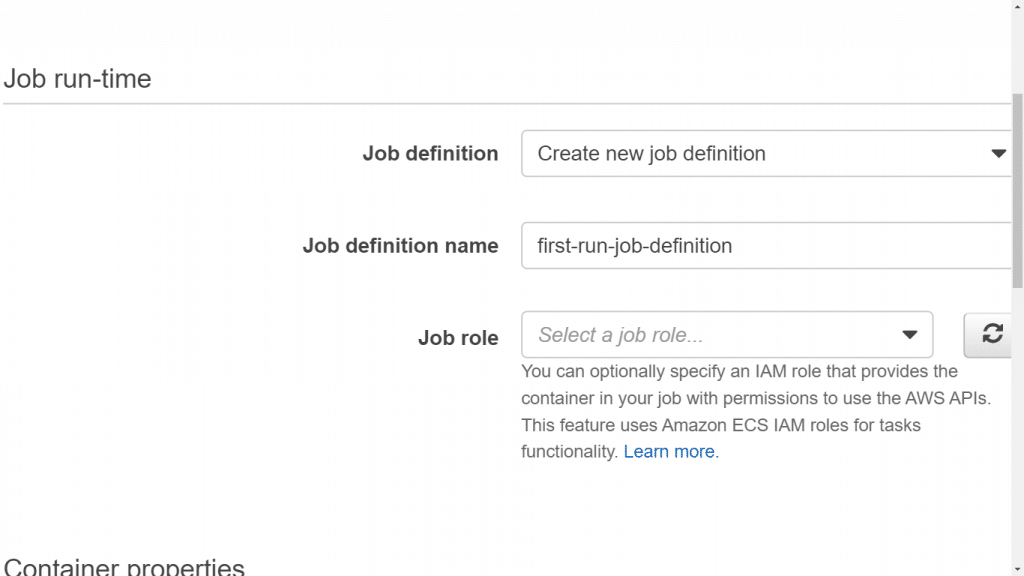This image captures a screenshot from a user’s device displaying a job configuration interface. The focus of the image is on a section labeled "Job runtime", which is followed by a faint gray line. Moving towards the middle and right side of the image, the section titled "Job Definition" is prominently displayed in black font. Below this, a white box outlined in gray includes the text "Create new job definition" and features a dropdown arrow indicating further options.

Further into the middle of the interface, the label "Job definition name" appears in black. In the corresponding input box, the text "first run job-definition" is visible. Directly below, another section labeled "Job role" contains the placeholder text "select a job role..." 

Beneath this, there is a gray informational paragraph explaining that users can optionally specify an IAM role, which provides the container within the job the necessary permissions to use AWS APIs. This feature leverages Amazon ECS IAM roles for task functionality. A "Learn more" hyperlink in blue is provided for additional information.

On the right side of the screenshot, a scroll bar is clearly visible. At the very bottom of the image, the text "Container properties" is partially visible, indicating another section related to job settings.